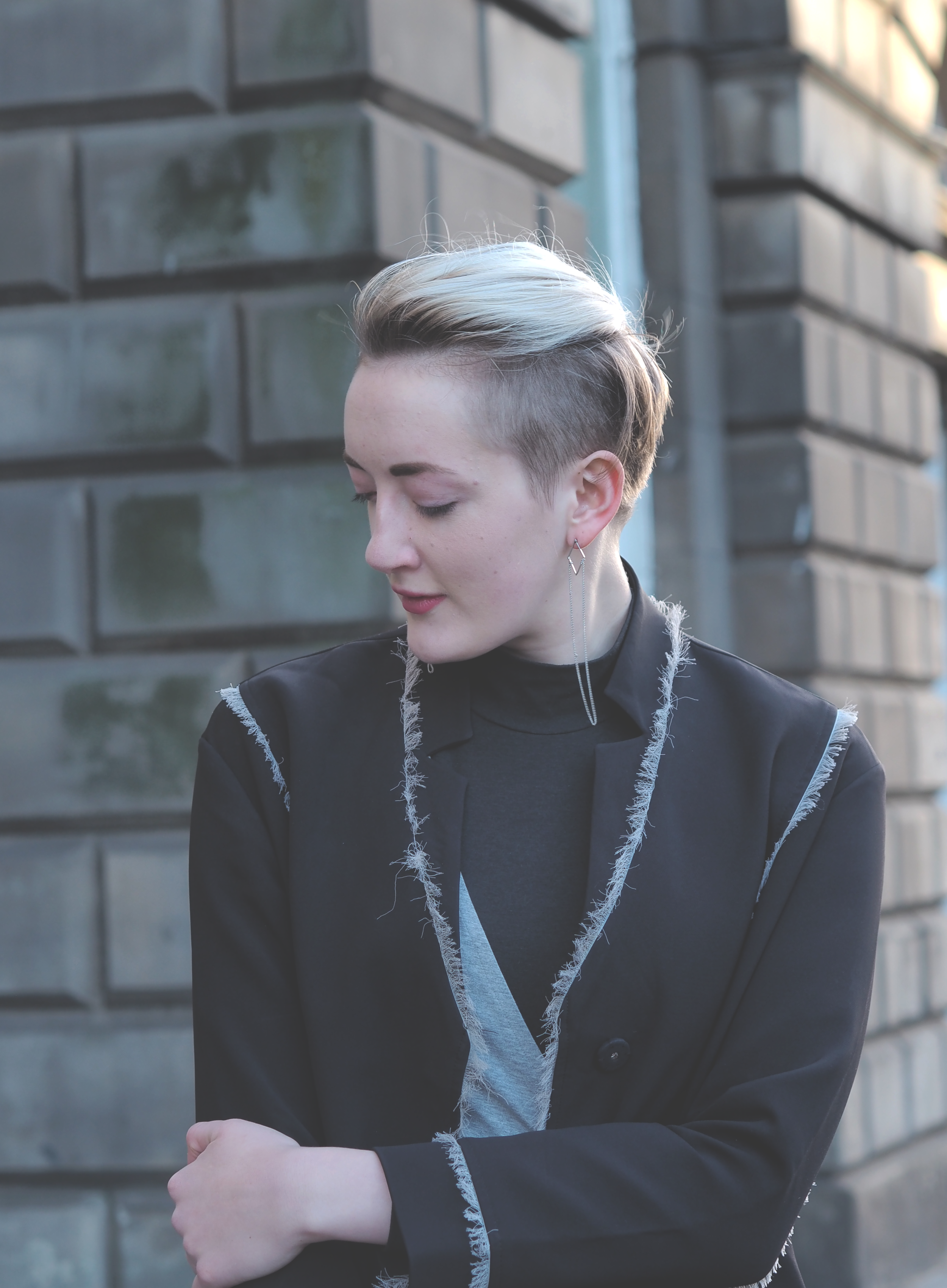The image captures a striking woman outdoors during the daytime, with a dull brown, brick building forming the backdrop. She is positioned in the center of the frame, gazing off to the left with her face in a slight side profile and her eyes closed, giving the impression of a contemplative or serene moment. Her distinctive hair is styled in a mohawk with the sides shaved, revealing a blend of blonde with darker undertones near the roots. She is adorned with long, gold earrings and has a black blazer featuring gray fringe along the seams. Under her blazer, she wears a black and gray turtleneck top. Her right hand is holding her left arm, adding a subtle, introspective gesture to her pose. Despite the possibility of studio lighting, the image strongly conveys the essence of natural daylight, adding to the authenticity and organic feel of the scene, which may hint at a fashion shoot or a magazine feature.